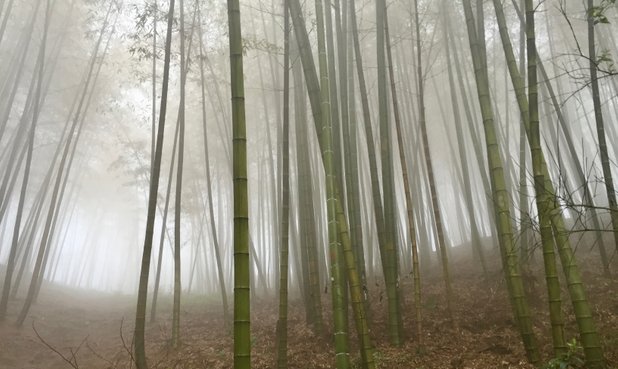This serene photograph captures the tranquil beauty of a bamboo forest shrouded in mist. The image features numerous tall, slender bamboo stalks rising straight from the ground to the top of the frame. The bamboo is segmented and exhibits a mix of green, silver, and black hues with distinct striations. As you gaze into the forest, the fog intensifies, especially towards the horizon, casting a bright white glow that gradually diminishes higher up. The canopy of the bamboo features leafy greenery, adding a touch of vibrancy to the scene. The forest floor is covered in a layer of brown leaves, suggesting a natural ground cover, likely consisting of fallen foliage. The overall setting is rural, with a muted color palette of greens, grays, silvers, and browns, contributing to the peaceful ambiance of this lush and expansive bamboo forest.